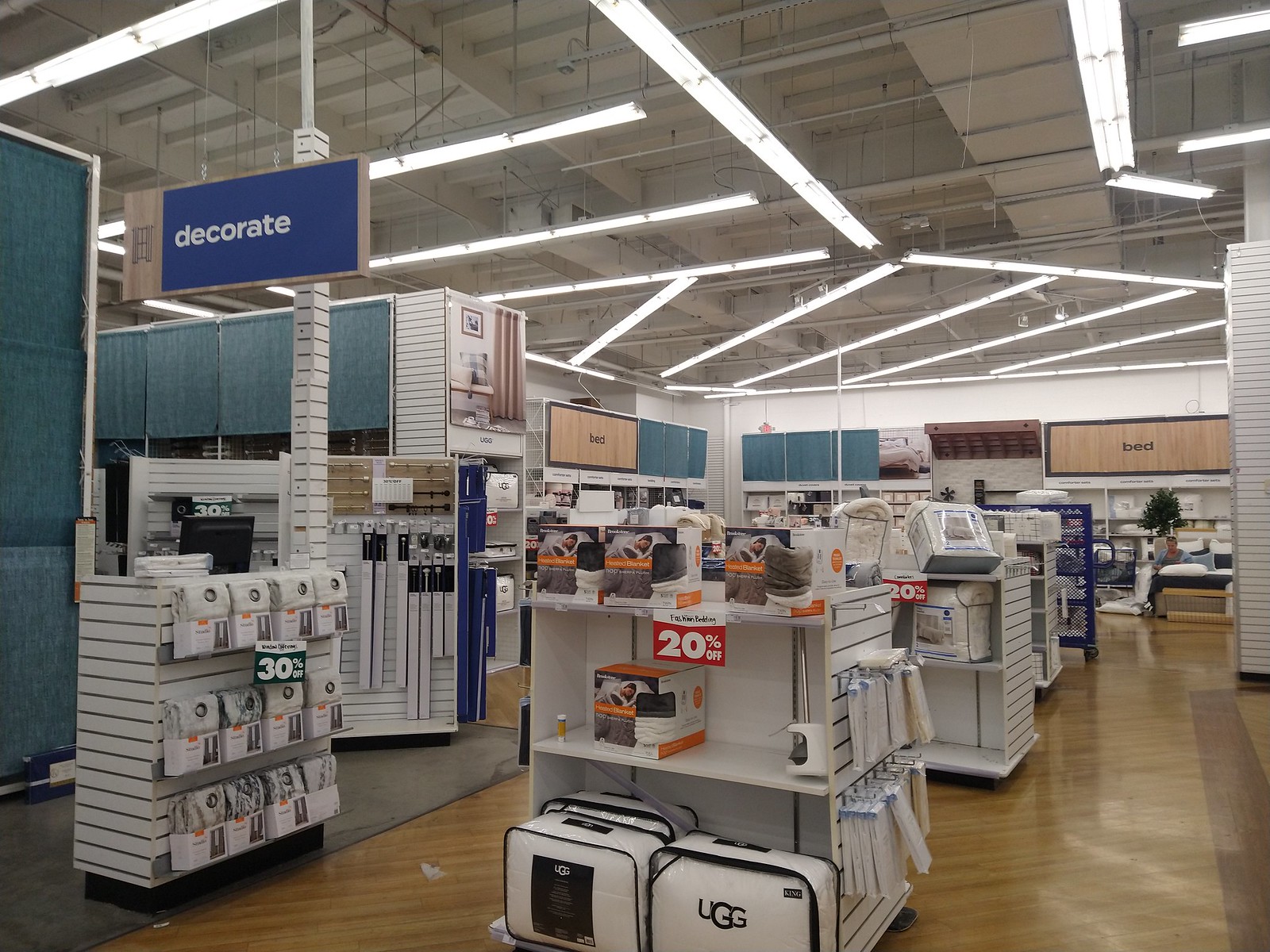The photograph captures the interior of a store, likely a Bed Bath & Beyond, specifically in the bedding section. The wooden floor leads the eye to various displays of bedding items. Prominent in the foreground, a bright red sign announces a 20% off sale on UGG-branded bedding, which is wrapped in see-through plastic packaging resembling small suitcases. Just to the left, a blue sign with white lettering reads "decorate," situated above shelves that possibly hold sheets or other decor items. In the background, several signs denote different aisles with a large brown "bed" sign prominently displayed above more bedding and comforters, and a green plant situated below it. The ceiling features exposed conduits, air conditioning vents, and long, bright rectangular fluorescent lights that illuminate the scene. Additionally, there are more shelves displaying a variety of products including towel racks and curtain rods. A woman can be seen seated on a bed towards the back of the store, adding a hint of human presence amidst the detailed, product-filled environment.